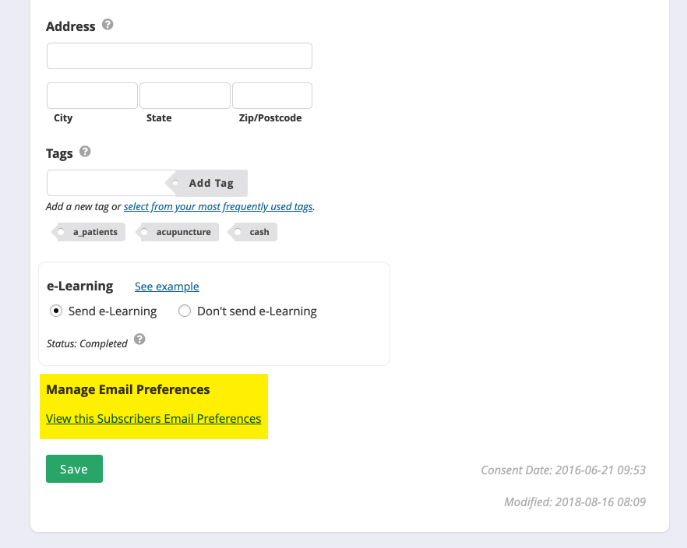"An interface displaying various input fields and settings for managing user information and preferences is shown. At the top, there are fields for entering an address, city, state, and zip/postcode. Below these fields, there's a section dedicated to tags, including a text box for inputting and adding tags. Users can either add a new tag or select from their most frequently used tags via a hyperlink labeled 'Select from your most frequently used tags'. Some of the tags listed include 'patient's acupuncture cache' and 'e-learning'. An example is provided with a hyperlink labeled 'see example here'. 

Further down, there are options for managing email preferences, with a checkbox to either 'Send e-learning' (which is currently checked) or 'Don't send e-learning'. The status of this setting is marked as 'Completed'. Additional options include hyperlinks labeled 'Manage email preferences' and 'View this subscriber's email preferences'. A green 'Save' button is available for saving changes. The interface also displays the 'Consent date' as June 21, 2016, at 9:53 AM, and 'Modified' date as August 16, 2018, at 8:09 AM."